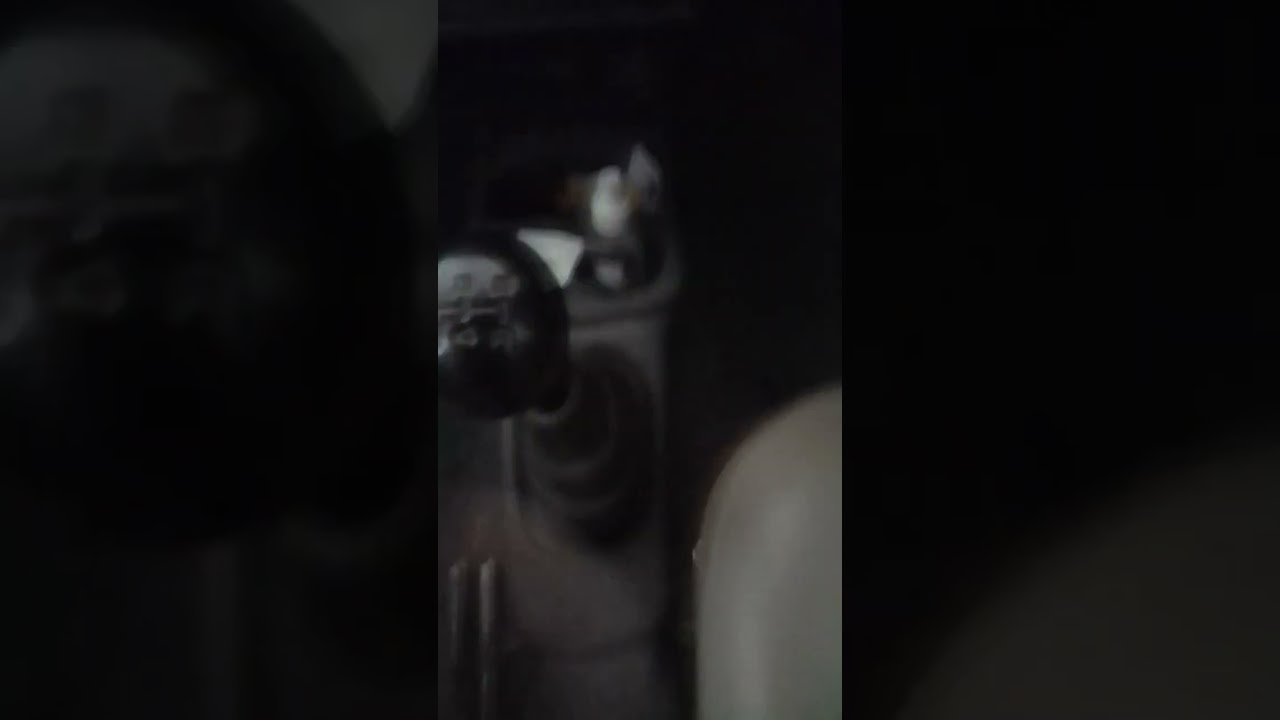The image is a grainy screenshot, reminiscent of a poorly captured moment from a mobile app like TikTok or Instagram Live. It is devoid of any text and primarily rendered in black, white, and various shades of gray, giving it a monochromatic and somewhat eerie appearance. The horizontal rectangular frame is flanked by black vertical stripes on either side, constraining the main content to the middle of the image. 

In the center, through the grain and blur, it appears to showcase a computer-generated or cartoon-like drawing of a man with gray skin. His face, turned slightly away, shows a visible eye and an open mouth, with a hand, likely his, emerging from the lower part of the image. The rest of his figure melds into the dark, almost black background, creating a stark contrast. Within this scene, there also seems to be a dark, shiny object protruding from what looks like a watering can, though the blurriness makes it ambiguous.

Upon closer inspection, the image might also be depicting an overhead view of a car's manual transmission console. The central figure could be interpreted as a gear shift knob, complete with a visible shifting pattern, set against an out-of-focus background resembling a car's interior panel. The overall scene, characterized by its indistinct and shadowy appearance, leaves many details open to interpretation due to the poor quality and high contrast of the colors.